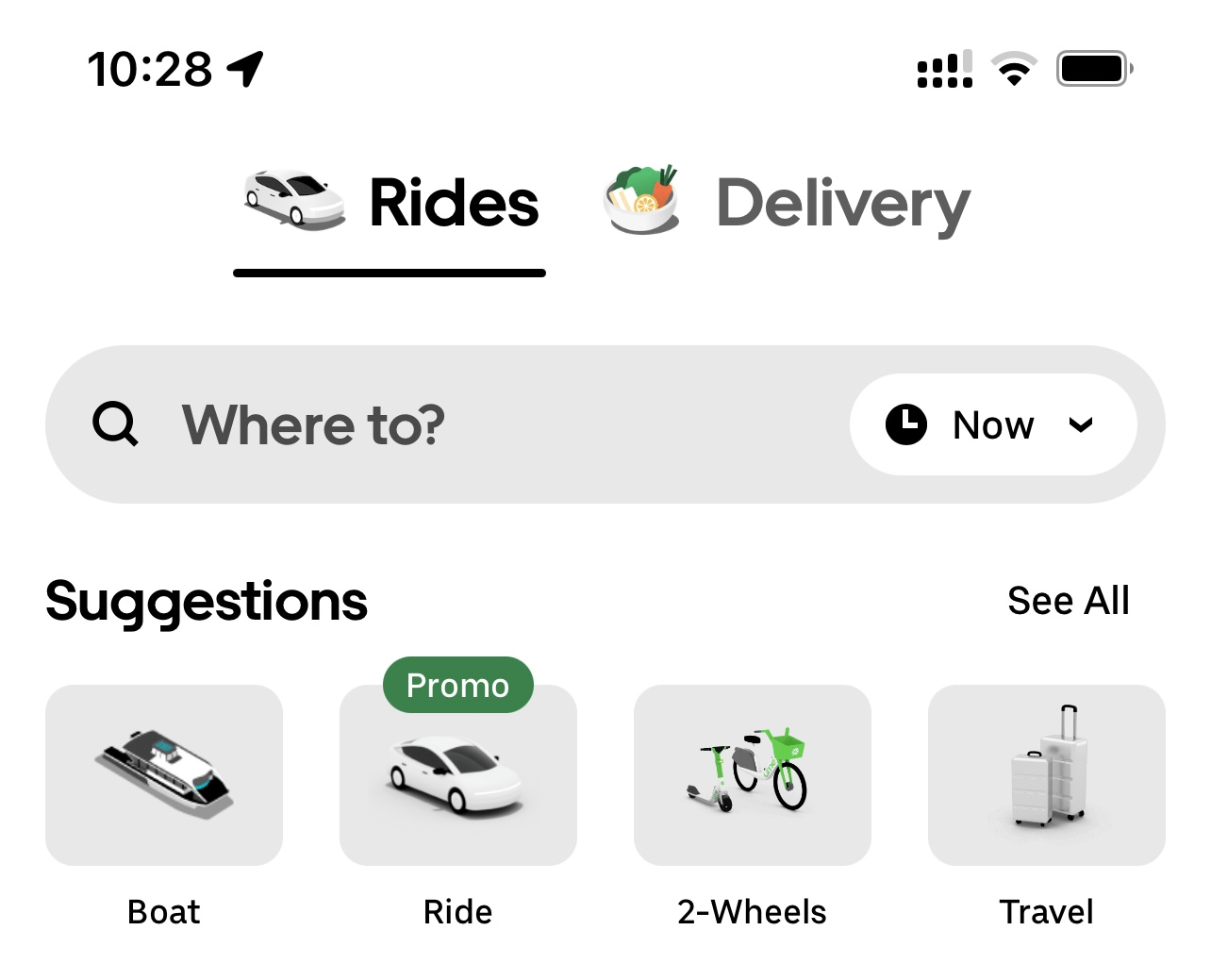This screenshot showcases a detailed view of a smartphone interface. At the top of the screen, the time is displayed as 10:28 on the left side, along with active location services and a notification status icon. On the right side, two network signal indicators are shown; the first indicates a signal strength of 3 out of 4 bars and the second a full signal strength of 4 out of 4 bars. The Wi-Fi icon is displayed next to a connected icon, and the battery level indicator is visible as well.

The main part of the page features two prominent sections: "Rides" and "Delivery." The "Rides" section is represented with an image of a car, while the "Delivery" section is illustrated with a picture of a ramen bowl. Other suggestions listed below include "Boats," "Ride," "Two Wheels," "Travel," and an option to "See All." Additionally, the right side has an active status section with a drum icon. There are no further details provided for this page.